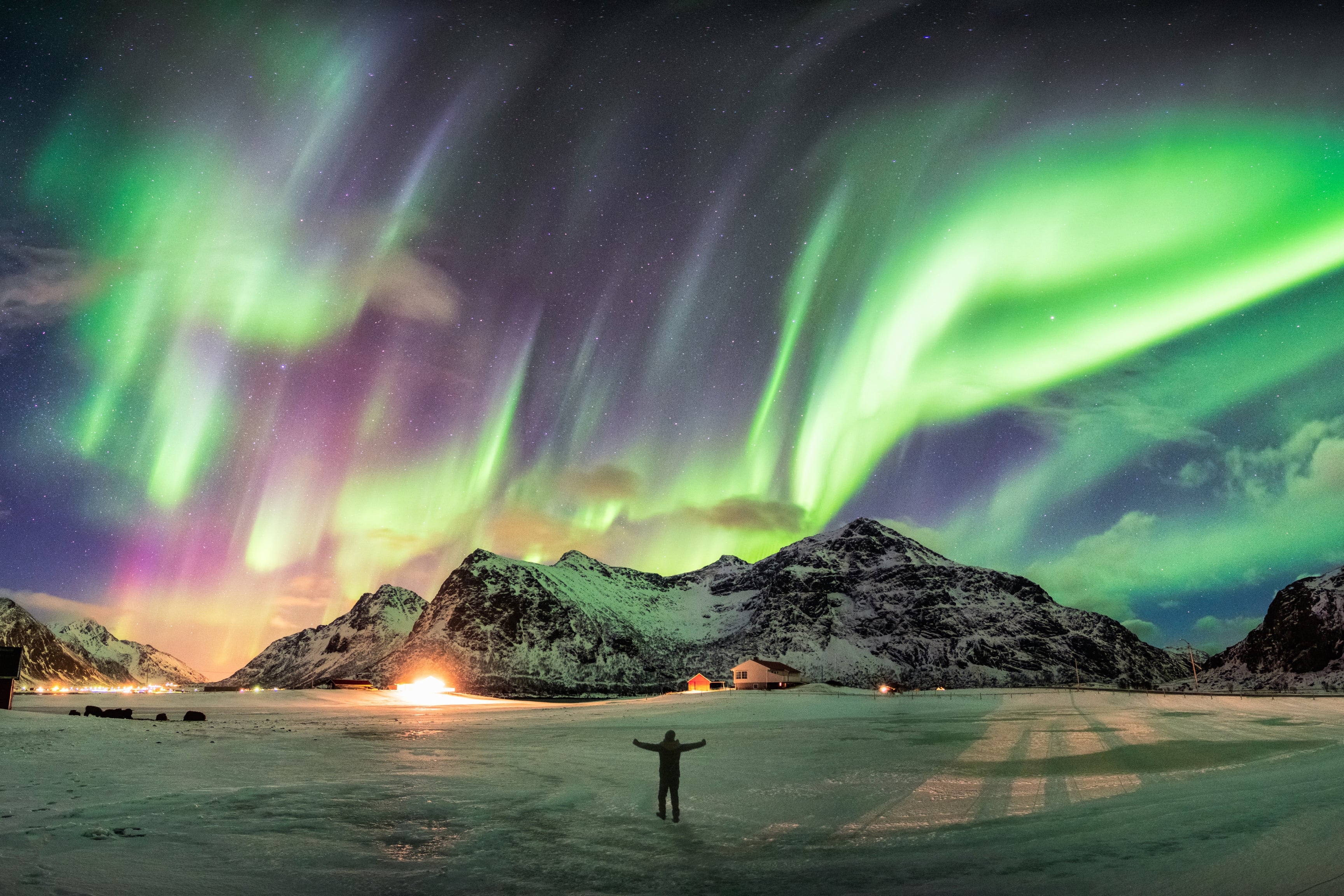In this computerized photograph, a solitary man stands centrally in an open, snowy field. His arms are outstretched, and he gazes ahead at a breathtaking scene, possibly set in a northern, mountainous region like Iceland, Greenland, or Alaska. Before him, a majestic, snow-capped mountain dominates the background, flanked by a two-story house and what appears to be a barn. In the distance, another car with lights further silhouettes the expansive scene. To the left of the man, a subtle glow suggests a distant fire or explosion, while further left, animals, perhaps bears, graze on the icy ground.

The vivid colors of the northern lights dance overhead, painting the sky in mesmerizing hues of green, yellow, dark and light purple, with accents of electric lime green and blue. These vibrant auroras contrast dramatically with the dark blue night sky. The landscape below, adorned with artificial yellow light from the sparsely positioned houses, fades into the monochrome of white snow and black mountain shadows. Clouds intersperse the light show, adding depth to the scene. The man’s dark clothing creates a stark silhouette against the luminous backdrop, embodying a moment of serene human connection with nature’s splendor in this meticulously detailed image.